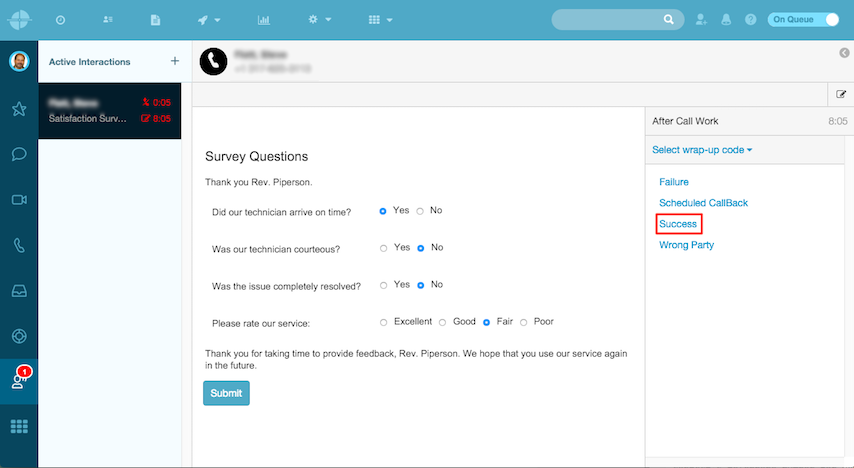This is a screenshot of a website with a light blue aesthetic. In the top left corner, there is a profile picture of a man with a receding hairline and a mostly bald head, smiling against a white background. To the right of his profile picture, the website displays "Active Interactions" indicating that he is currently in a call. The call has only been active for five seconds, which suggests he either has the person on hold or the call recently concluded.

In the top section of the screen, the name and number of the person he is calling are blurred out, but a phone icon is visible next to the obscured details. At the bottom of the screenshot, there are survey questions that imply the call has ended. The survey begins with a thank you message addressed to "Rev Piperson," followed by several questions about the recent service interaction. The questions and responses are:

- "Did our technician arrive on time?" Answer: Yes.
- "Was our technician courteous?" Answer: No.
- "Was the issue completely resolved?" Answer: No.
- "Please rate our service?" Answer: Fair.

These responses reveal that the individual did not have a satisfactory experience with the service.